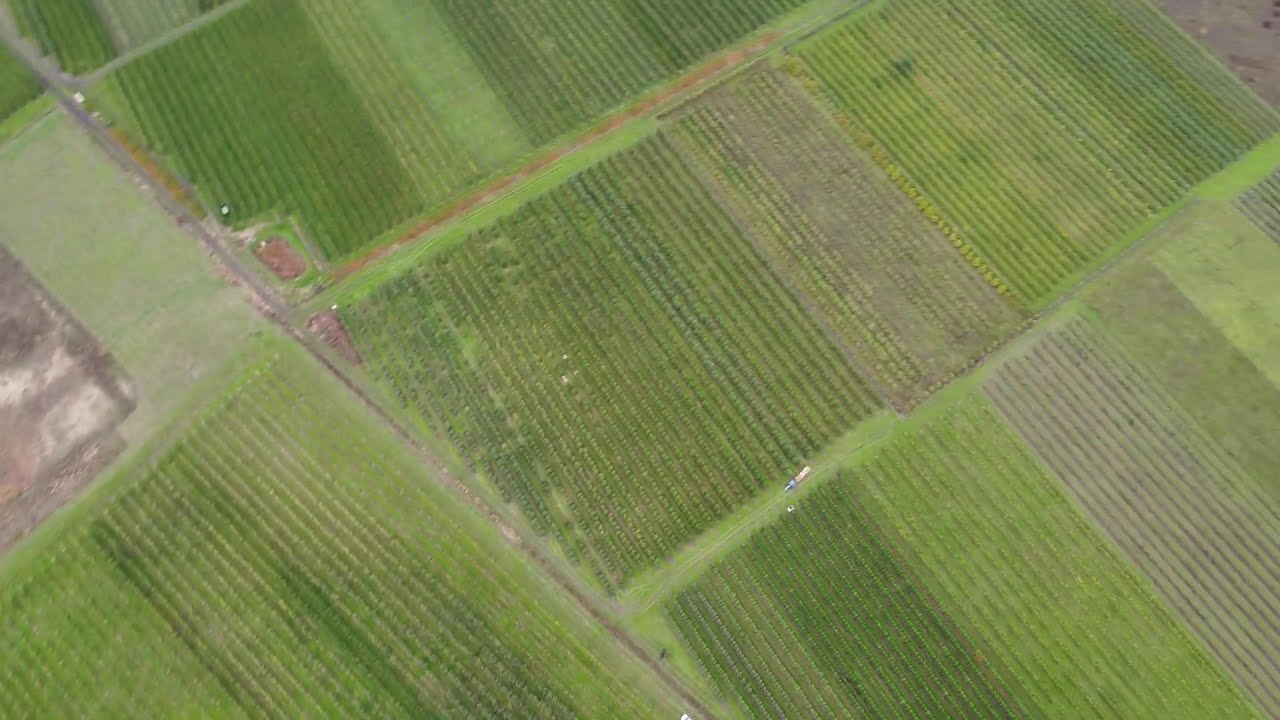The image is an overhead aerial view of a farmland agricultural landscape captured from a few hundred feet above. The expansive field is sectioned into about nine distinct parcels, presenting a contrasting checkered pattern of varying shades of green and brown. The rows of crops predominantly stretch from the lower right to the upper left, creating an angled orientation across the land. Among the vibrant green patches, there are also areas of bare dirt and lighter beige, suggesting recently excavated plots or fallow sections.

In the left-center of the image, a gray dirt area disrupts the consistent green, possibly indicating a turnout or a garden. A discernible dirt road or path meanders from the middle-bottom, angling towards the upper left of the photo, bisecting the farmland into left and right segments. To the left of this path, two parcels stand out – one with a lighter green color at the top potentially indicating a structure, the other with densely organized crop rows. A couple of smaller paths run parallel to the main road, further dividing the green expanse into agricultural sections.

There's a small, indistinct speck near the dirt area that could be a person wearing a light-colored shirt or hat, though it isn't clear enough to confirm. Similarly, a tiny vehicle, possibly with a trailer, is faintly visible towards the middle bottom of the image, positioned within one of the dirt paths between sections. The scene is devoid of any visible buildings, and the predominant colors are green and brown, with no readable text or sky in sight.